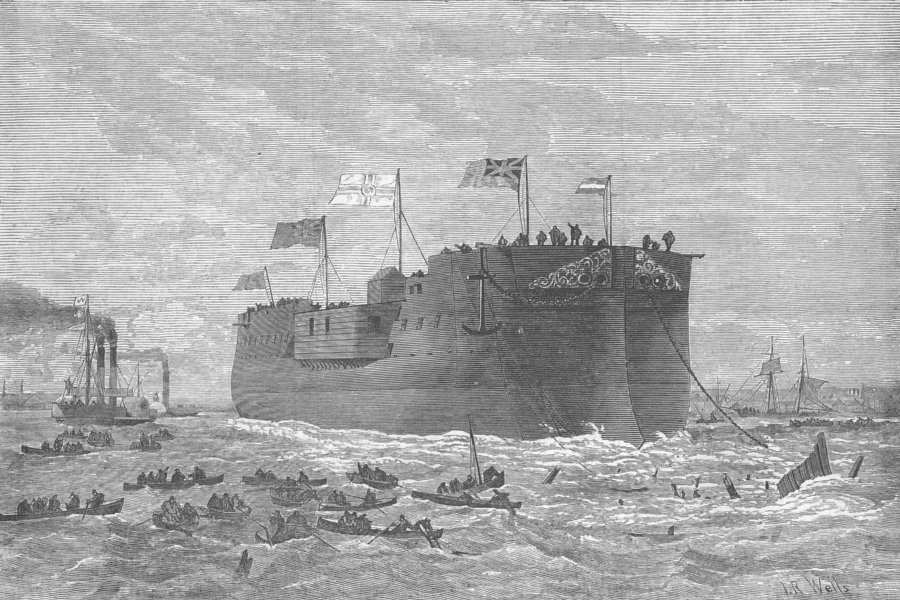The image is a detailed, black and white illustration of a colossal, wooden warship navigating through choppy, gray waters. The ship, towering over everything in the scene, dominates approximately 30% of the image and features multiple flags—five in total—each with distinct designs, distributed along its tall structure. Hanging over the sides are anchors, and a line of about ten men is visible at one of the large openings on the ship. Surrounding this majestic vessel are several smaller lifeboats and rowboats, filled with people struggling to stay afloat amidst the turbulent waves. The waves are depicted with intense white crests, crashing dynamically against the ship's hull. To the right side of the image, smaller sailboats and steamships, significantly dwarfed by the massive warship, can be seen. The sky above is dense with fluffy yet heavy clouds, contributing to the dramatic and somber atmosphere of the scene.